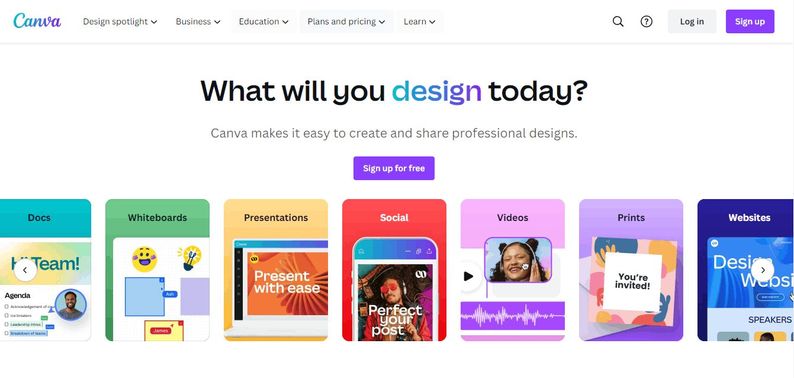A detailed screenshot of the Canva website is presented, showcasing the user-friendly interface and various design options it offers. The webpage features a clean, predominantly white background with a faint, almost imperceptible light gray line separating the top menu from the main content area.

In the upper left corner, the recognizable Canva logo is visible, styled in an elegant script. The "CAN" portion of the logo is in a pleasant sky blue, while the "VA" is in a rich purple. To the right of the logo, a series of gray-font menu items are listed: "Design," "Spotlight," "Business," "Education," "Plans and Pricing," and "Learn," each followed by an inverted triangle, indicating drop-down menus.

On the upper right side of the header, a prominent purple rectangle with white text invites users to "Sign Up." Adjacent to it, a light gray rectangle with darker gray text offers a "Login" option. To the left of the login button, there is a gray-outlined circle with a gray question mark, likely serving as a help or information resource. Further left, the gray search icon is depicted as a circle with a line extending from its lower right, resembling a magnifying glass.

The main headline, centered on the page in bold black font, poses the question, "What will you design today?" Notably, the word "design" is uniquely colored to match the Canva logo, with "DES" in light blue and "IGN" in purple. Beneath this headline, a subheading in gray font states, "Canva makes it easy to create and share professional designs."

Below the subheading, a central purple rectangle with white text encourages users to "Sign Up for Free." Under this call to action, a series of vertical rectangles in various colors represent different types of design categories. Each rectangle features a distinct colored top border and a label: "Docs" (blue), "Whiteboards" (green), "Presentations" (light orange), "Social" (red), "Videos" (light lavender), "Print" (purple), and "Websites" (blue). Each rectangle includes a small sample of design elements relevant to its category, illustrating the diverse tools and templates Canva offers to its users.